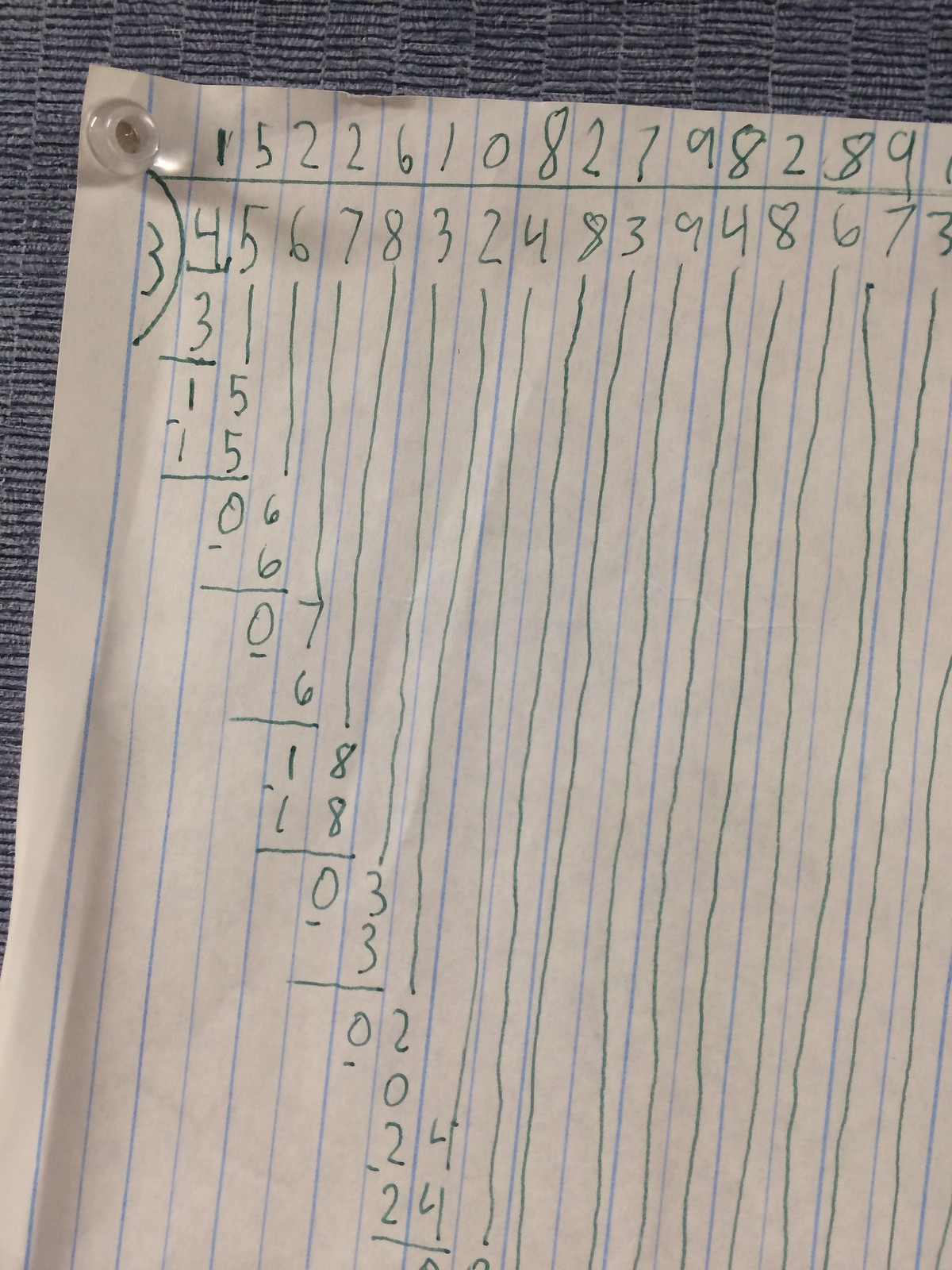The image features a piece of lined paper, oriented vertically, with the lines running top to bottom instead of the usual horizontal format. The paper is light blue, accentuated with blue lines, and is attached to a gray fabric-like board using a clear push pin at the top center. The push pin secures the paper, which seems to display a complex math problem.

Across the top of the paper, written in green ink between each line, is a series of numbers: 1, 5, 2, 2, 6, 1, 0, 8, 2, 7, 9, 8, 2, 8, 9. Directly below these numbers, a green line is drawn horizontally across the paper.

Beneath this line, still in green ink, the first noticeable number is 3, enclosed within a bracket at the back. Following this 3 is a sequence of numbers: 4, 5, 6, 7, 8, 3, 2, 4, 8, 3, 9, 4, 8, 6, 7, 3. Immediately below the initial 4, the next significant number 3 has a line underneath it. To the right of this 3, there is the number 1, followed by 5. Below this 1 and 5 pairing, there is another set of 1 and 5, also underlined. Finally, under the bottom-most 5, the number 0 is written.

The overall appearance of the image suggests meticulous detail and precision as the person works through the math problem, showcasing an intricate array of numbers and notations.